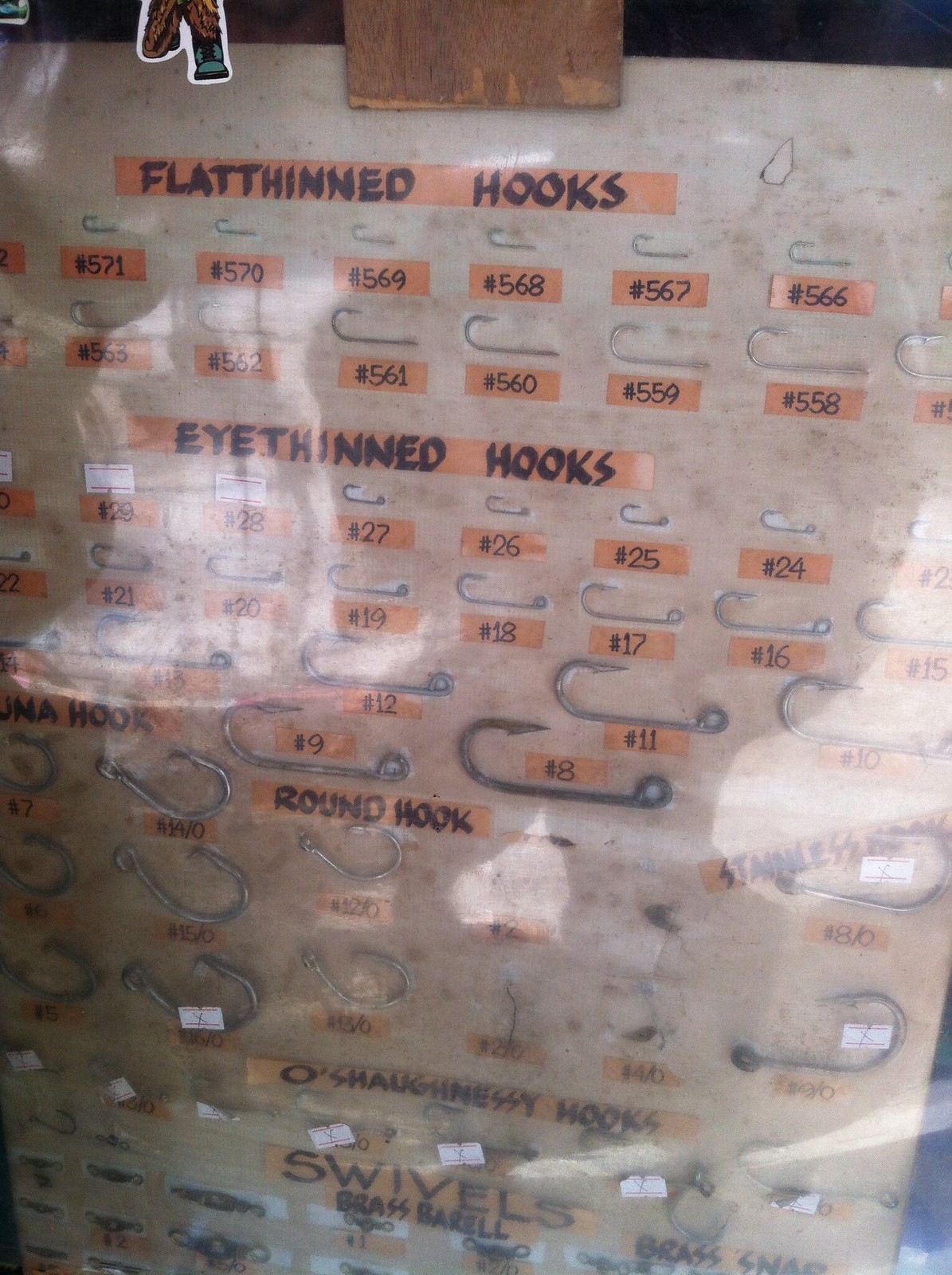This photographic image captures a detailed display of various fish hooks, likely seen in a hardware or sporting goods store. The hooks are meticulously arranged on a white board, possibly made of cardboard, which is encased in a reflective plastic sheet. This gives the appearance of viewing the display through a glass window. Each hook is distinctly catalogued with an orange Scotch tape label, featuring numbers that help identify the different types, including flat-thinned hooks, eye-thinned hooks, round hooks, O'Shaughnessy's hooks, and swivels. The assortment spans a wide range of sizes, from tiny to extra-large, exemplifying the diverse options available for fishing enthusiasts. The display's meticulous organization and clear labeling ensure that customers can easily select and order hooks based on their desired specifications.